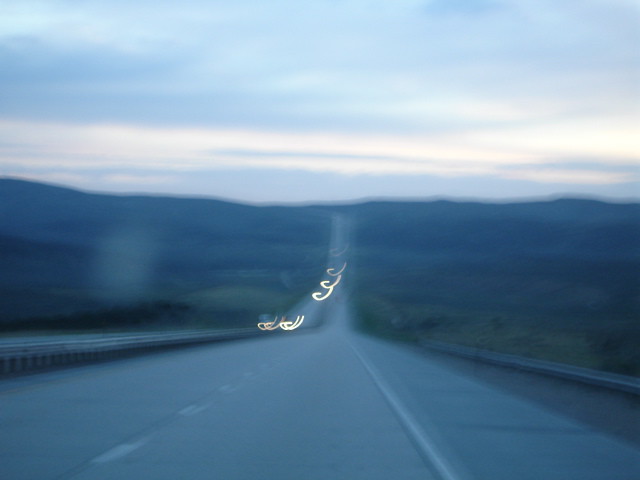The image depicts a scene of a winding roadway descending a hill, characterized by a blue-dominated color palette. The asphalt appears to have an unusual blue hue, possibly due to the prevailing lighting conditions or image processing. A dotted white line in the center indicates a two-way traffic flow, while substantial guardrails line both sides of the road, ensuring safety on this potentially treacherous descent.

On the right side, there is a sizable emergency lane, clearly marked and ready for use if needed. Although no individual vehicles are discernible, there's a dynamic swirl of white lights on the opposing side of the road, suggesting oncoming traffic. The background and sky blend into various shades of blue, interspersed with wisps of white clouds, contributing to the surreal quality of the scene. 

The surrounding landscape features soft, rolling hills that are primarily olive green but subtly transition into the overarching blue theme. The roadway, framed by these blended hues, stretches straight down the middle of the image, leading towards a distant horizon where it appears to flatten out and possibly rise again, suggesting an undulating terrain.